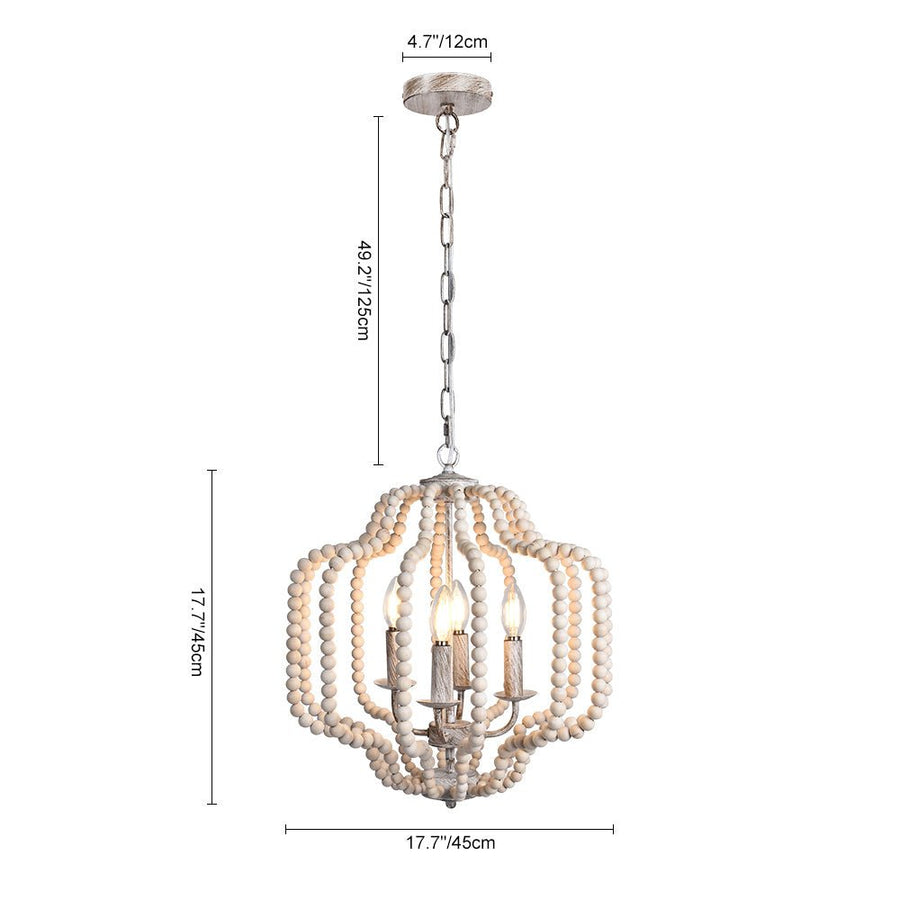The image depicts a chandelier suspended against a white background, focusing solely on the fixture detailed with dimensions. The chandelier features four candle-shaped lights centered within a unique structure composed of large, pebble-like beads that are stacked and spaced to reveal the light. The overall design of the beaded formation around the lights gives the chandelier a somewhat squared appearance. It hangs from a chain measuring 49.2 inches (125 cm) in length. The top portion of the chandelier is 4.7 inches by 12 centimeters. The midsection of the chandelier, encompassing the lighting structure itself, measures 17.7 inches (45 cm) in both height and width. The detailed diagram includes various markings, elucidating the measurements of each component of the chandelier.